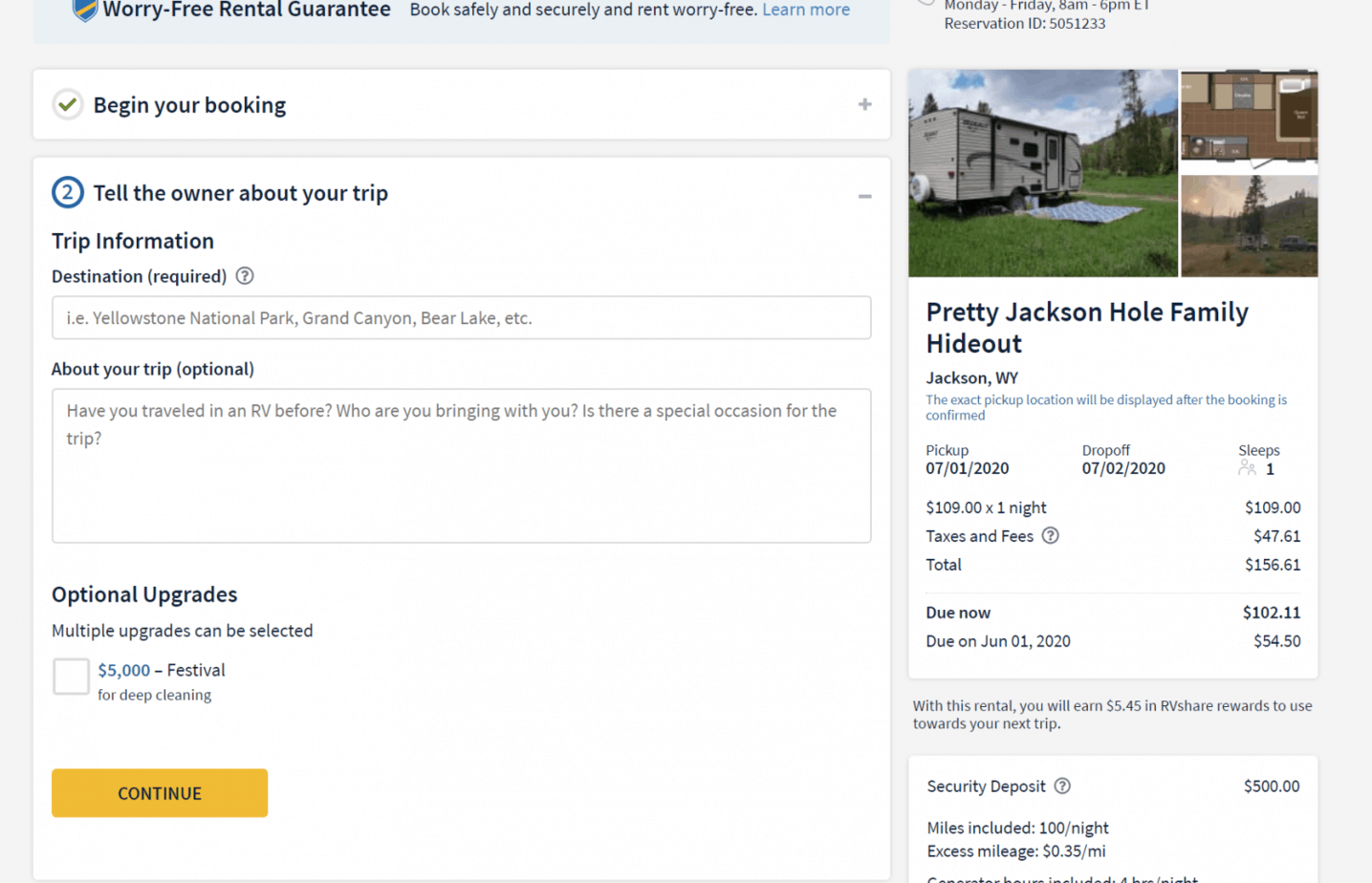This image is a detailed screenshot of a booking confirmation for a stay at a residence. At the top of the screenshot, a banner prominently displays the message "Worry-Free Rental Guarantee: Book Safely and Securely, Worry-Free." An additional prompt reads "Learn More," suggesting further information is available. The business hours, listed as Monday through Friday, 8 a.m. to 6 p.m. ET, are clearly visible. The reservation ID, which is 505-1233, is also displayed.

On the top left of the image, a section titled "Begin Your Booking" is marked. Underneath, a white input box prompts users to "Tell the Owner About Your Trip." Within this box, fields such as "Trip Information" and "Destination (Required)" encourage users to input destinations like "Yeltsin National Park, Grand Canyon, Bear Lake, etc." There is also an optional section labeled "About Your Trip," which asks, "Have you traveled in an RV before? Who are you bringing with you? Is there a special occasion for the trip?"

Below this, another section titled "Additional Upgrades" offers multiple selectable upgrades, including a $5,000 festival package and deep cleaning services. A prominent golden button with black text labeled "Continue" is displayed for advancing the booking process.

On the right-hand side of the image, more specific reservation details appear. This includes a couple of images showcasing a camper and a scenic outdoors area with green hills and trees, illustrating the serene environment. The caption underneath the images describes the destination as "Pretty Jackson Hole Family Hideout in Jackson, Wyoming." It is noted that the exact pick-up location will be revealed once the booking is confirmed. The financial details indicate that the person paid $109 for one night, and after adding taxes and fees, the total cost amounts to $102.11. A partial payment of $54.50 is due on June 1, 2020.